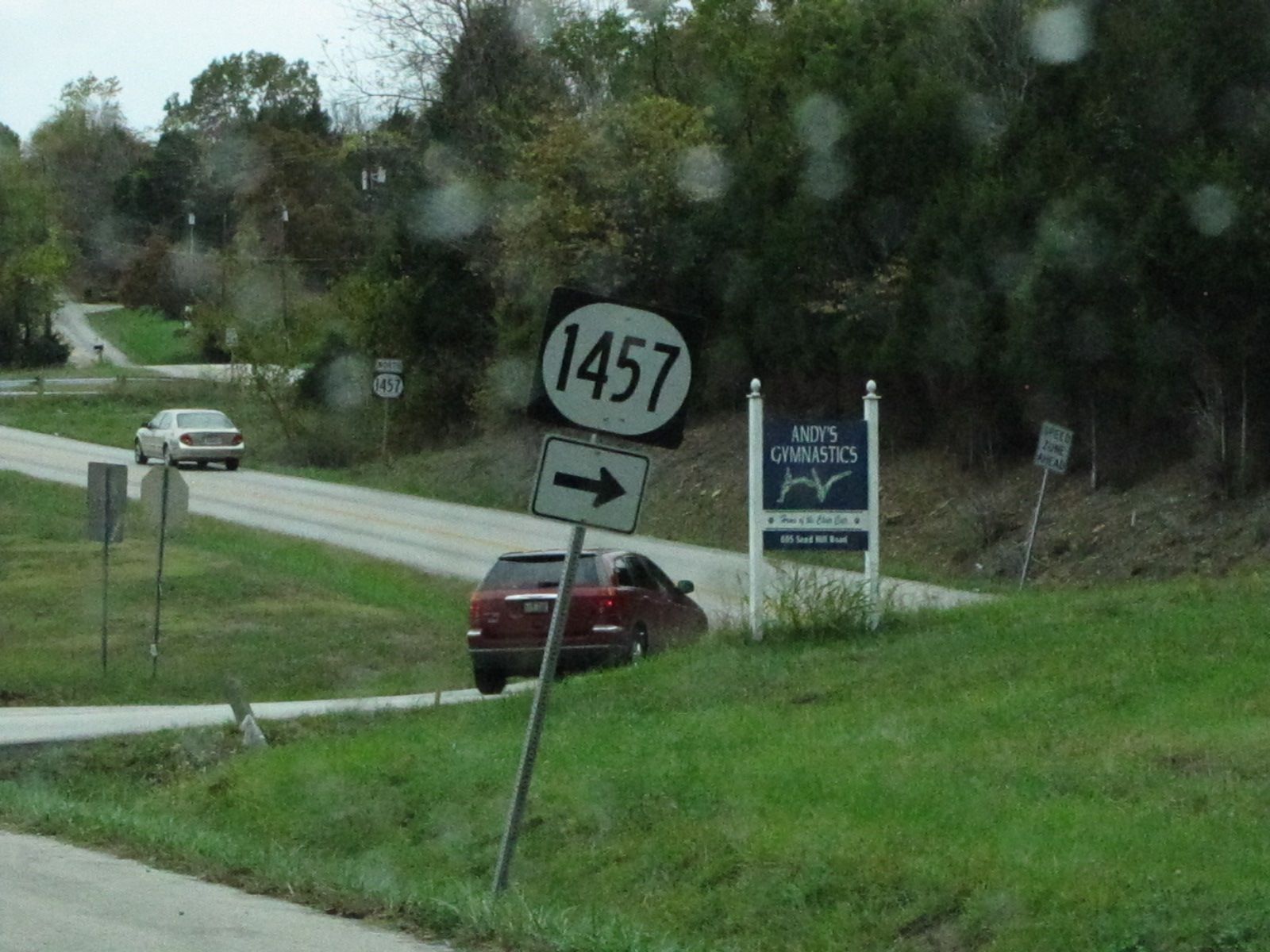The image depicts a private road surrounded by lush greenery and hilly terrain, illuminated by a light faded gray asphalt surface. Prominently featured are two vehicles: a red car in the center and a whitish-silver car in the background, both traveling in the same direction. Numerous signs punctuate the scene, including a black-and-white route number 1457 sign with an arrow pointing to the right and another indicating a "Speed Zone Ahead." A navy and white sign advertising "Andy's Gymnastics" stands out among the roadside scenery. Additional details include visible power poles, side roads, other street signs seen from behind, and a possible mailbox on the top left. The backdrop is dominated by clusters of leafy green trees and overgrown grass, painted with a few blurry, cloudy circles that add a layer of textured ambiance to the image.